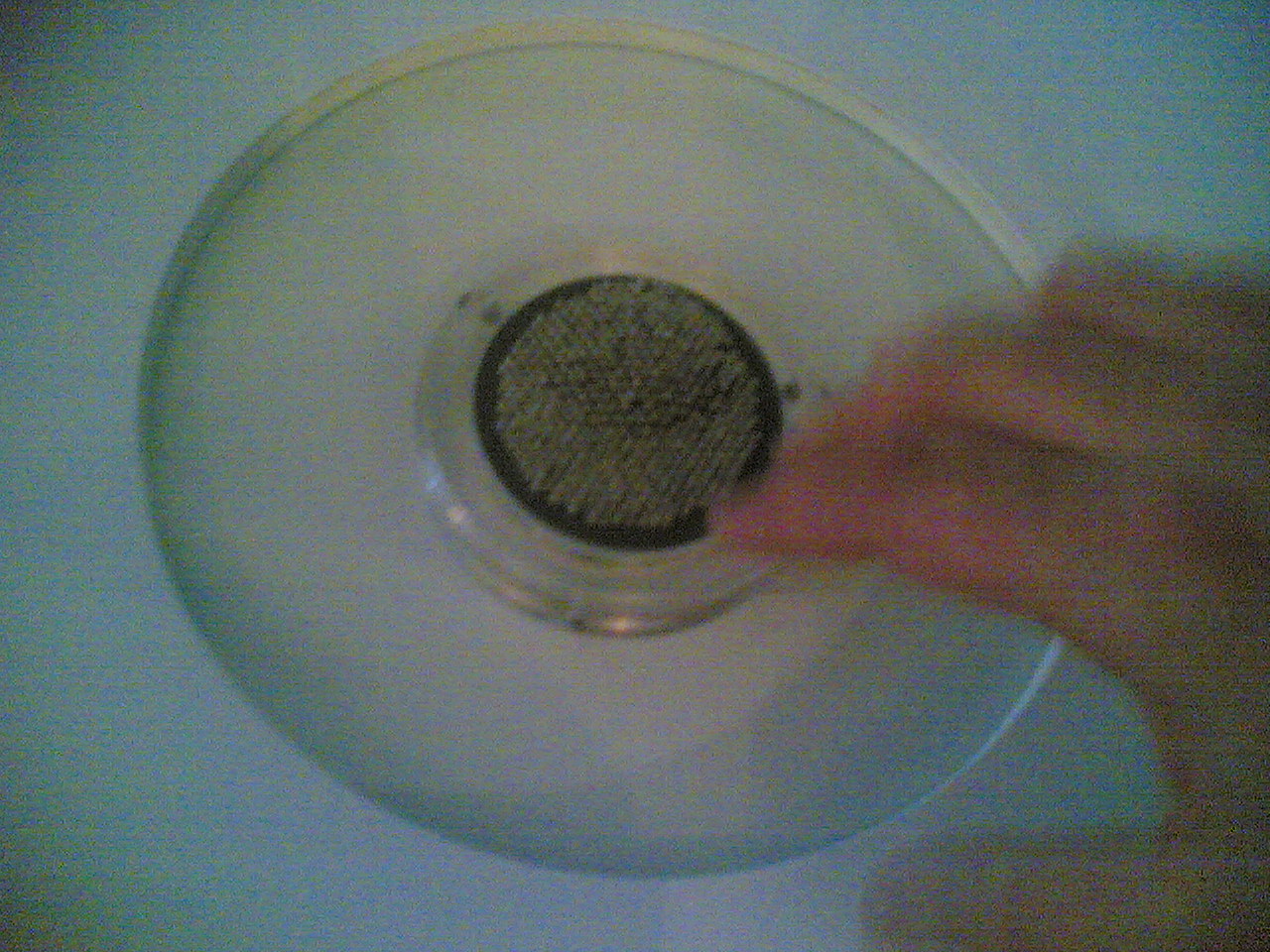This image depicts a circular object, possibly photographed indoors on a white surface with blue coloration around the edges. The centerpiece is a transparent circular glass dish that houses a smaller, intricate black disc in the middle, which appears to be made up of numerous pin-sized holes or dots, resembling pin needle heads. Surrounding the black disc is another white circle, possibly a plastic holder, which gives the entire setup a layered circular appearance. The scene shows signs of age and some blurriness, especially evident in the background and along the edges. On the left side of the image, a hand with a visible thumb and three fingers reaches towards the central black area, adding a touch of interaction and scale to the composition. This intricate setup could belong to a light fixture, a drain, a speaker, or a laboratory device, indicated by the organized circular strata and the presence of what might be dust or dirt in the middle.